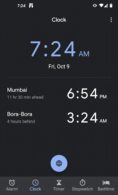The image features a black background with multiple digital time displays and icons. At the top, the screen prominently shows the time "7:24 AM" in purple, and below it, the date "Friday, October 4th" in white. Beneath this, there are additional time zones listed: "Merto - 6:54 AM" and "Bora Bora - 3:24 AM," both displayed in white text. Central to the image is a large purple circle with a smaller black circle inside it. At the bottom of the screen, there is a row of icons—an airplane, a clock, a timer, and two others that are slightly blurry and difficult to discern. The display effectively showcases the local time alongside times in two other locations.